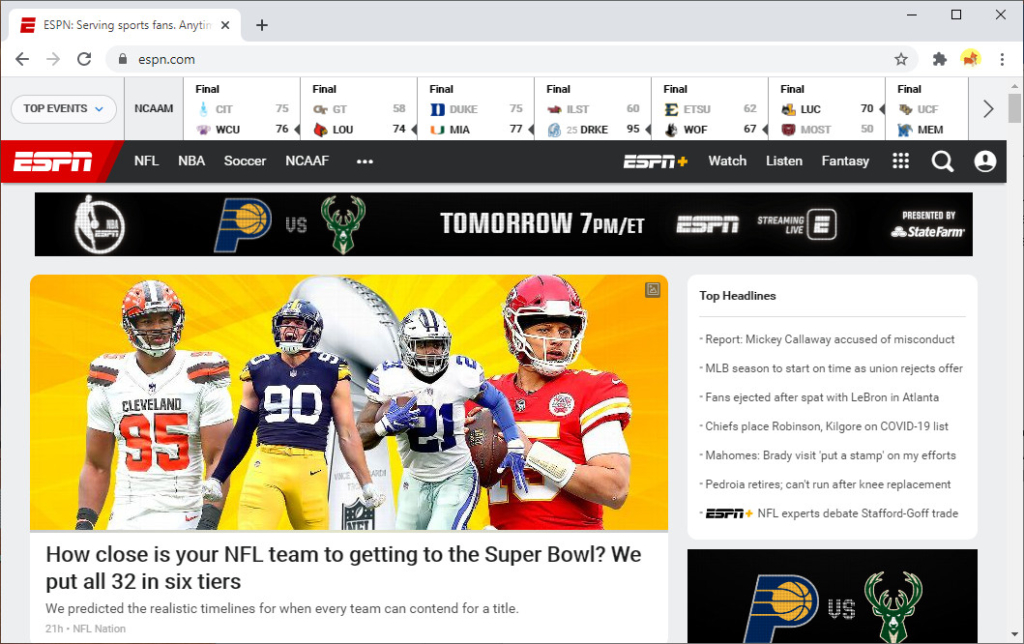This is a screenshot of an ESPN webpage with a clean and structured layout against a light gray background. In the upper left corner, the browser tab features the ESPN emblem—a red "E"—followed by black text reading "ESPN: Serving Sports Fans." 

Directly below is the ESPN search bar for easy navigation. The page continues with a section labeled "Top Events," accompanied by a dropdown menu. This section displays several finalized sports match results listed as follows:
- NCAA.am (Final: CIT 75 - WCU 76)
- GT 58 - LOU 74 (Final)
- Duke 75 - MIA 77 (Final)
- ILST 60 - DRKE 95 (Final)
- ETSU 62 - WOF 67 (Final)
- LUC 70 - MOST 50 (Final)
- UCF vs. MEM (Final, with a directional arrow pointing to the right).

Beneath this, a white "ESPN" logo sits prominently on a bold red background. This is followed by a long black bar featuring navigation links in white text, including "NFL," "NBA," "Soccer," and "NCAAF."

The center of the page showcases an image of four football players from different teams. Underneath the image, an insightful caption reads: "How close is your NFL team to getting to the Super Bowl? We put all 32 in six tiers. We predicted the realistic timelines for when every team could contend for a title."

To the right side of the main image, a section is dedicated to listing the top headlines, providing quick access to the latest sports news.